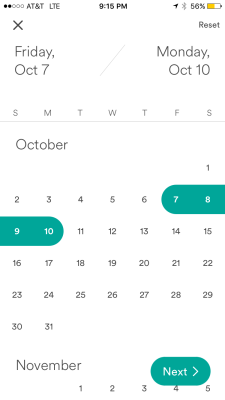This image captures a detailed screenshot of an iPhone displaying a calendar month view for October, with the top status bar indicating the phone is in Low Power Mode at 56% battery life, signified by the yellow battery icon. The iPhone is connected to the AT&T network and is currently operating on LTE. The time displayed is 9:15 PM, although the exact year is not specified.

The calendar view is minimalistic, featuring a white background and thin, gray text. Notably, the dates from Friday, October 7th to Monday, October 10th are highlighted in green, suggesting a period of importance. Additionally, the interface shows part of the upcoming month, specifically the first five days of November. Below the battery indicator, there is a "Reset" button, and a green "Next" button, which might seem redundant considering the calendar already highlights a green date range within October.